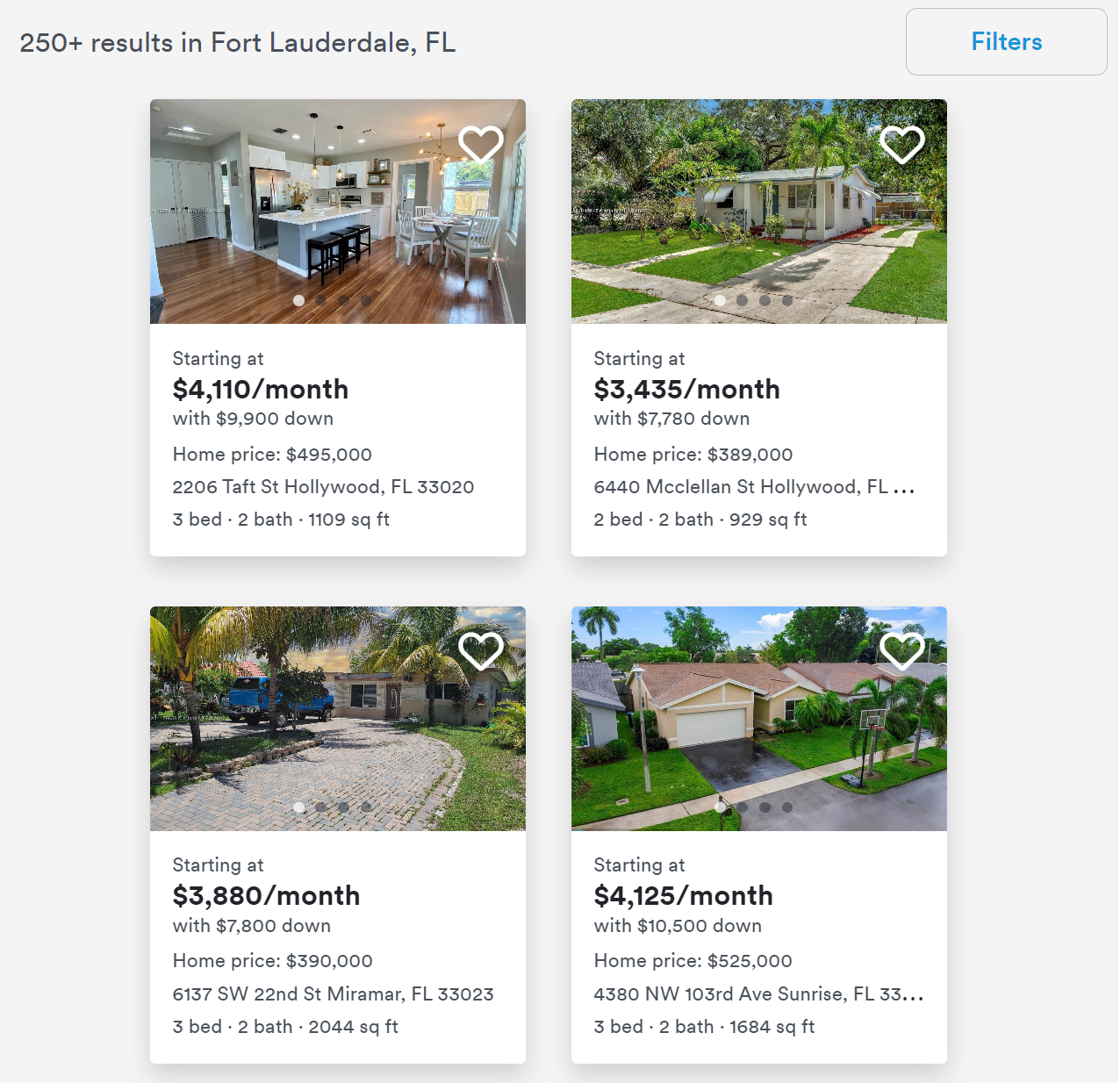The image features a detailed display of four house listings arranged in a 2x2 grid, each illustrated with an image and accompanied by comprehensive details. At the top of the image, a header notes "250+ Results in Fort Lauderdale, Florida," while a blue "Filters" button is situated in the upper right corner.

**Top Left Listing:**
- **Image Description:** Features a modern kitchen adjoining a main living area.
- **Price:** Starting at $4,110 a month.
- **Down Payment:** $9,900.
- **Additional Information:** Listed below the image are the home price, address, number of bedrooms and bathrooms, and square footage.

**Top Right Listing:**
- **Image Description:** Displays an exterior view of a cozy white ranch-style house.
- **Price:** Starting at $3,435 a month.
- **Down Payment:** $7,780.
- **Additional Information:** The home is priced at $389. Additional details include the address, two bedrooms, two bathrooms, and 929 square feet of space.

**Bottom Left Listing:**
- **Image Description:** Shows an exterior view of a small ranch-style house surrounded by palm trees.
- **Price:** Starting at $3,880 a month.
- **Down Payment:** $7,800.
- **Additional Information:** This home features three bedrooms, two bathrooms, and spans 2,044 square feet.

**Bottom Right Listing:**
- **Image Description:** Displays an exterior view of another small ranch-style house.
- **Price:** Starting at $4,125 a month.
- **Down Payment:** $10,500.
- **Additional Information:** It includes three bedrooms, two bathrooms, and covers 1,684 square feet.

Overall, these listings offer a variety of housing options in Fort Lauderdale, showcasing different styles, sizes, and price points, aimed at providing potential buyers with detailed and organized information.